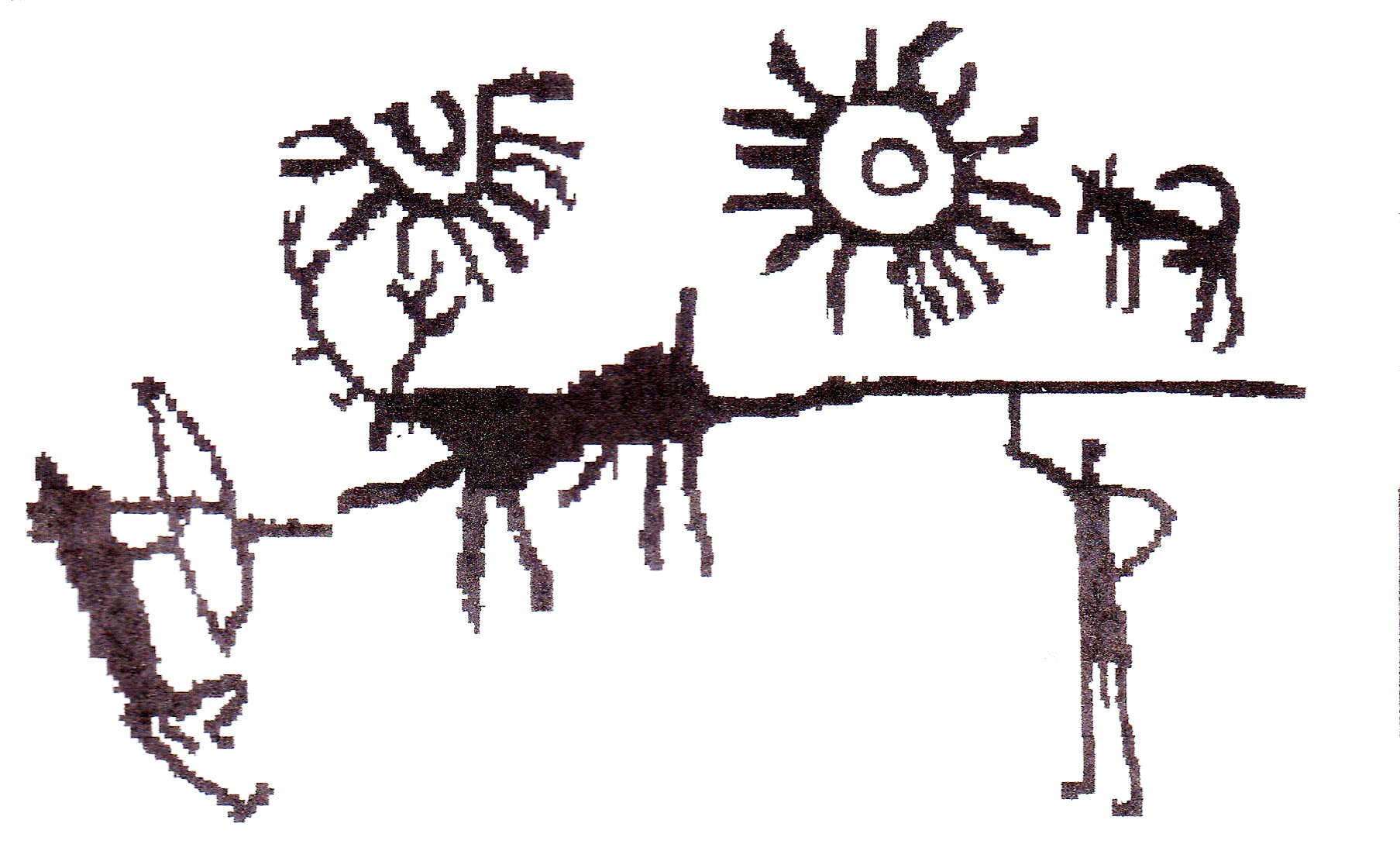The image is a pixelated drawing that captures a primitive or indigenous style illustration, potentially telling a hunting story. It is set on a white background with the figures presented in black and brown pixels. On the far left, a human figure holds a bow and arrow, aiming at a deer or an elk with prominent antlers located towards the center-right of the scene. This deer stands on a horizontal line that signifies the horizon. Above the deer, there is an ambiguous pixelated shape that might represent a bird. Nearby, another human figure, possibly wielding a spear, appears below the horizon line. In the top right, there is an animal that resembles a monkey, depicted on all fours with a tail. Next to it is a stylized sun with concentric circles and rays emanating outward. This intricate and pixelated depiction seems to narrate an ancient hunting expedition.